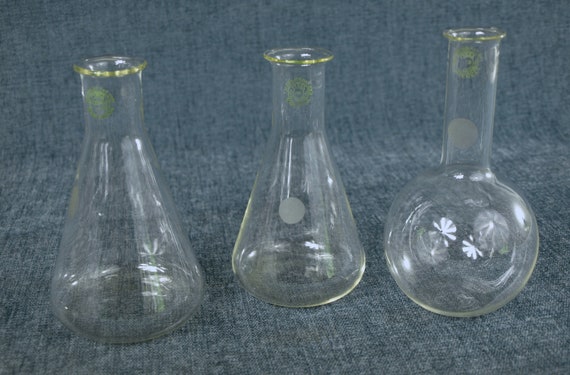The image features three distinct flasks positioned on a deep blue or dark cloth surface that extends up behind them. The first two flasks on the left and in the middle share a similar design: a flat, round bottom that narrows upward and then extends straight up to a fluted rim, with a gold trim around the top. The flask on the far right diverges in shape, characterized by a long neck leading to a large, bulbous bottom, also adorned with a gold rim. The beakers are transparent, and embellished with small gold stamps or stickers; the center flask has a circular sticker, while the flask on the right has stickers with half-sun or floral designs near the opening. All three flasks are empty, allowing a clear view through them.